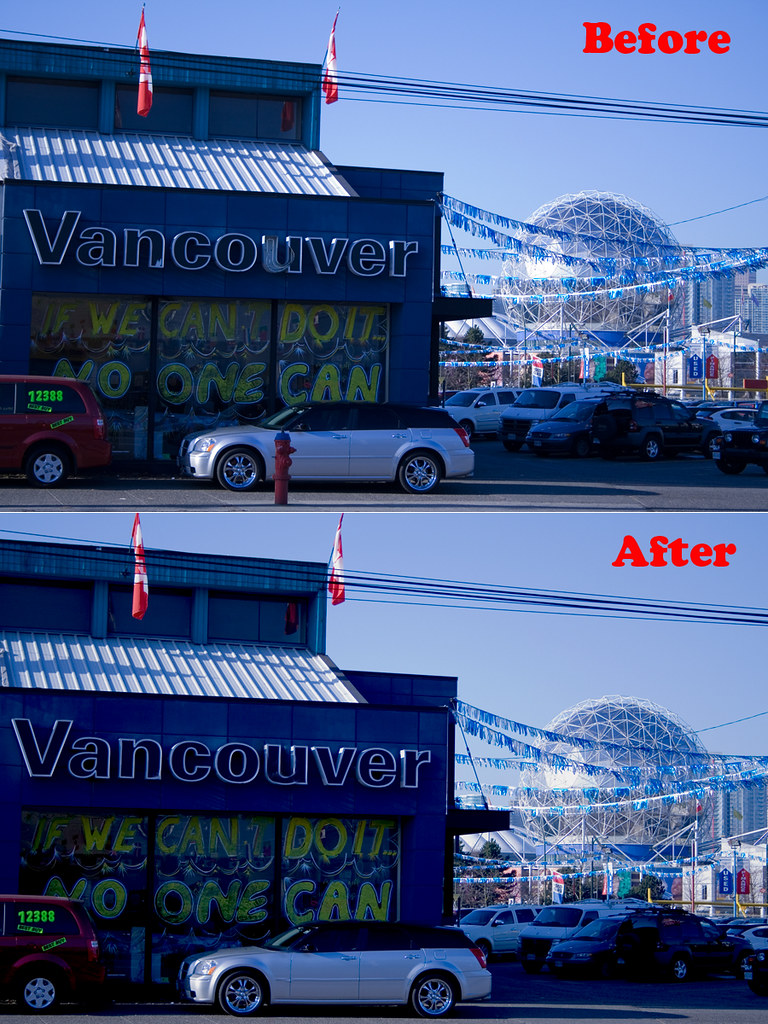The image consists of a before-and-after comparison set outside what appears to be a car dealership. The top part, labeled "before" in red text in the top right corner, shows a building with a damaged sign reading "Vancouver," where the "U" is falling apart. The building has an awning over the sign and features a second floor set slightly back. Canadian flags are flying over the structure, and the windows display the slogan, "If we can do it, if we can't do it, no one can." In front of the building, there are multiple parked cars, with one car on the left displaying the number "12388" on its window, likely indicating a price. There are stickers on this car as well. A big blue dome-shaped display with a crisscross pattern of white bars forming triangles and octagons is visible in the background, and strings with little flags or ribbons drape across the scene, adding a festive touch. Notably, a fire hydrant is present in the foreground of this image.

In the bottom part, labeled "after," the scene is almost identical but taken slightly later in the day. The crucial difference is the "Vancouver" sign, which has been repaired, with all letters, including the previously damaged "U," now looking intact and uniform. The fire hydrant seen in the first photo is missing in this one. Otherwise, the arrangement of cars, the building’s appearance, and other details remain the same, emphasizing the repair of the sign as the significant change between the "before" and "after" shots.